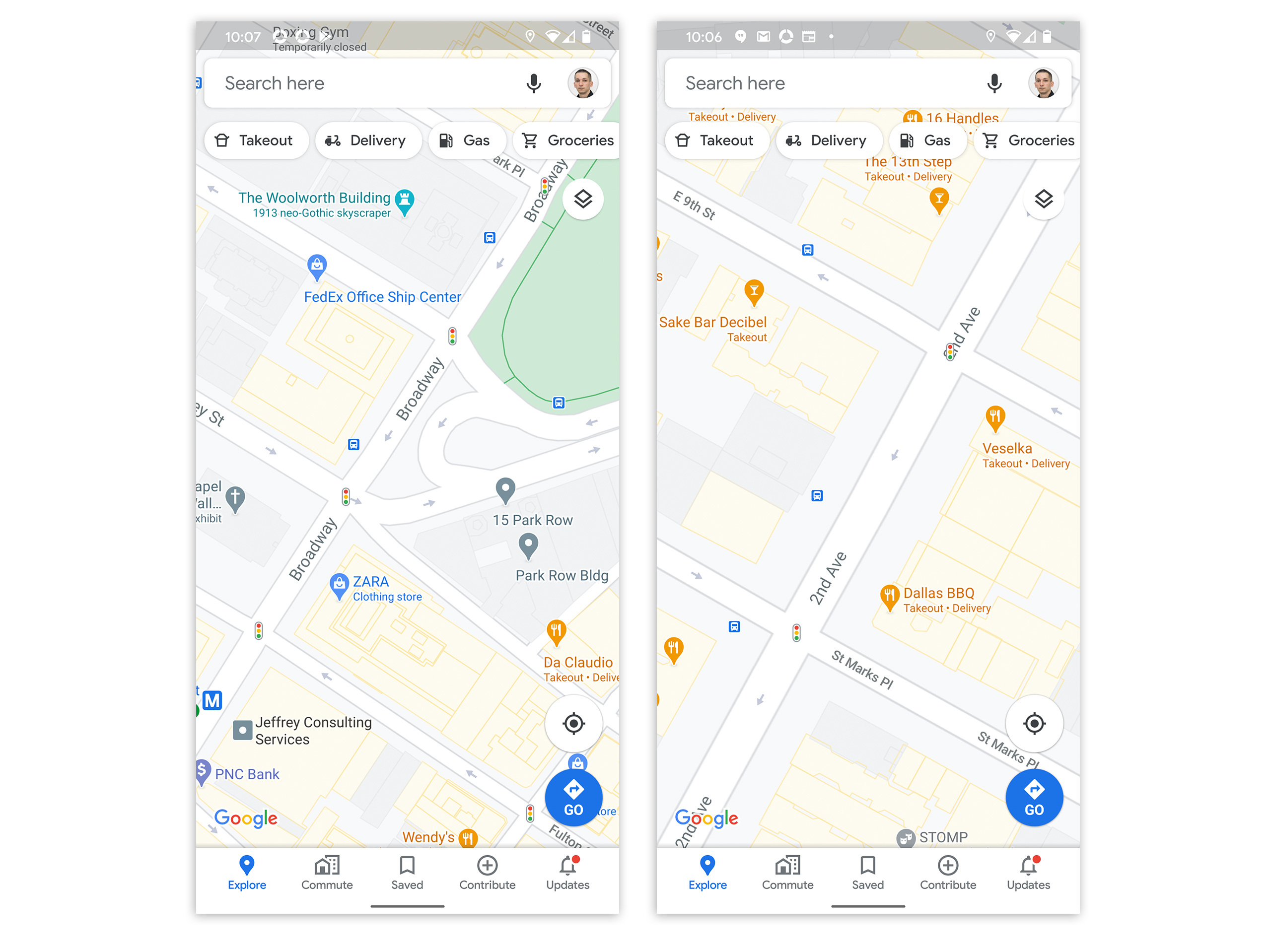The image displays two side-by-side screenshots from a mobile device, both taken from Google Maps. 

In the left screenshot, the time is 10:07 AM. There is a Google Play Store notification, indicating some activity or update. The device shows poor Wi-Fi and phone signals, while the battery level appears mostly charged. The "Search here" field in Google Maps is empty. Beneath it are quick-access options such as "Takeout," "Delivery," "Gas," and "Groceries." The profile picture in the top-right corner features an image of a white man, consistent across both screenshots. The displayed map highlights notable landmarks such as the Woolworth Building, a 1913 Neo-Gothic skyscraper, Zara, Wendy's, Broadway Street, and the lower corner of a park.

In the right screenshot, the time is 10:06 AM, marked by an email push notification. Like the left screenshot, the "Search here" field remains empty, and the same profile picture is visible. The quick-access options under the search field also include "Takeout," "Delivery," "Gas," and "Groceries." The map differs, showcasing streets and landmarks including 2nd Avenue, 9th Street, St. Mark's Place, and establishments such as Sake Bar Decibel, Veselka, Dallas Barbecue, and The 13th Step.